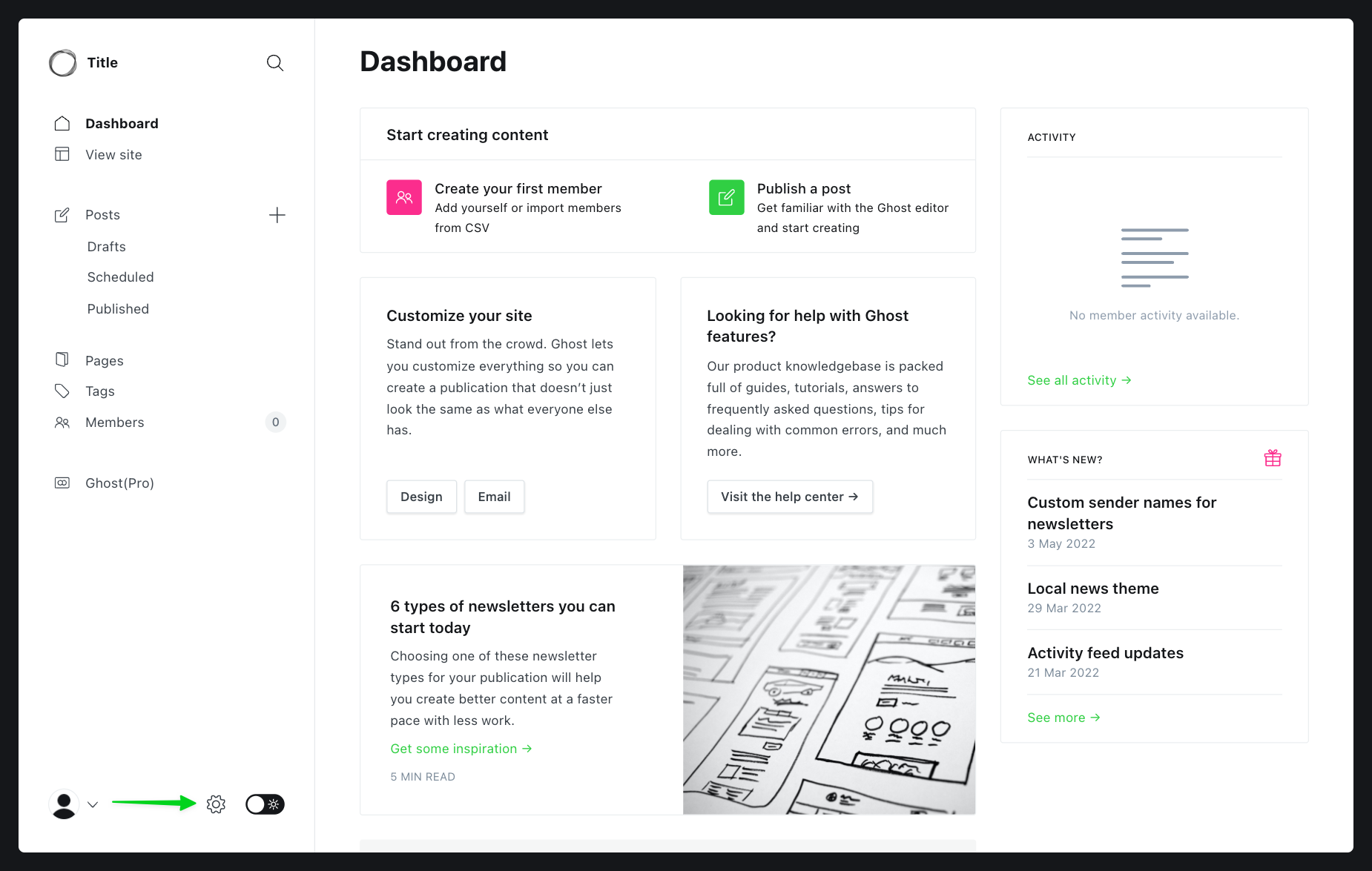The image depicts a webpage interface that appears to be from a content management system, likely designed for website editing and blogging. The page has a white background and is framed by a prominent black border. The layout is approximately 30% to 50% wider than it is tall. 

On the left-hand side, there is a vertical navigation menu. At the top of this menu is a title section followed by several clickable options with accompanying icons:
- "Dashboard," with a house icon,
- "View Site," with a window icon,
- "Posts," with an edit icon,
- "Drafts," "Scheduled," "Published," "Pages," "Tags," and "Members," each without icons,
- "Ghost (Pro)" at the bottom, with no icon but "Pro" enclosed in parentheses.

To the right of the navigation menu is the main content area. At the top of this section, aligned to the left in bold text, is the label "Dashboard". Below this heading is a prompt encouraging the user to start creating content. Specific callouts include:
- A section labeled "Create your first member," with further details instructing users to "add yourself or import members from CSV". This section is accompanied by a pink square icon featuring two people.
- Another section prompting users to "Publish a post," aimed at familiarizing them with the Ghost editor to begin creating. To the left of this section is a green box with an "Edit" button.

The overall design suggests a user-friendly interface intended for managing and publishing web content, likely meant for users who are setting up or managing a blog or website.